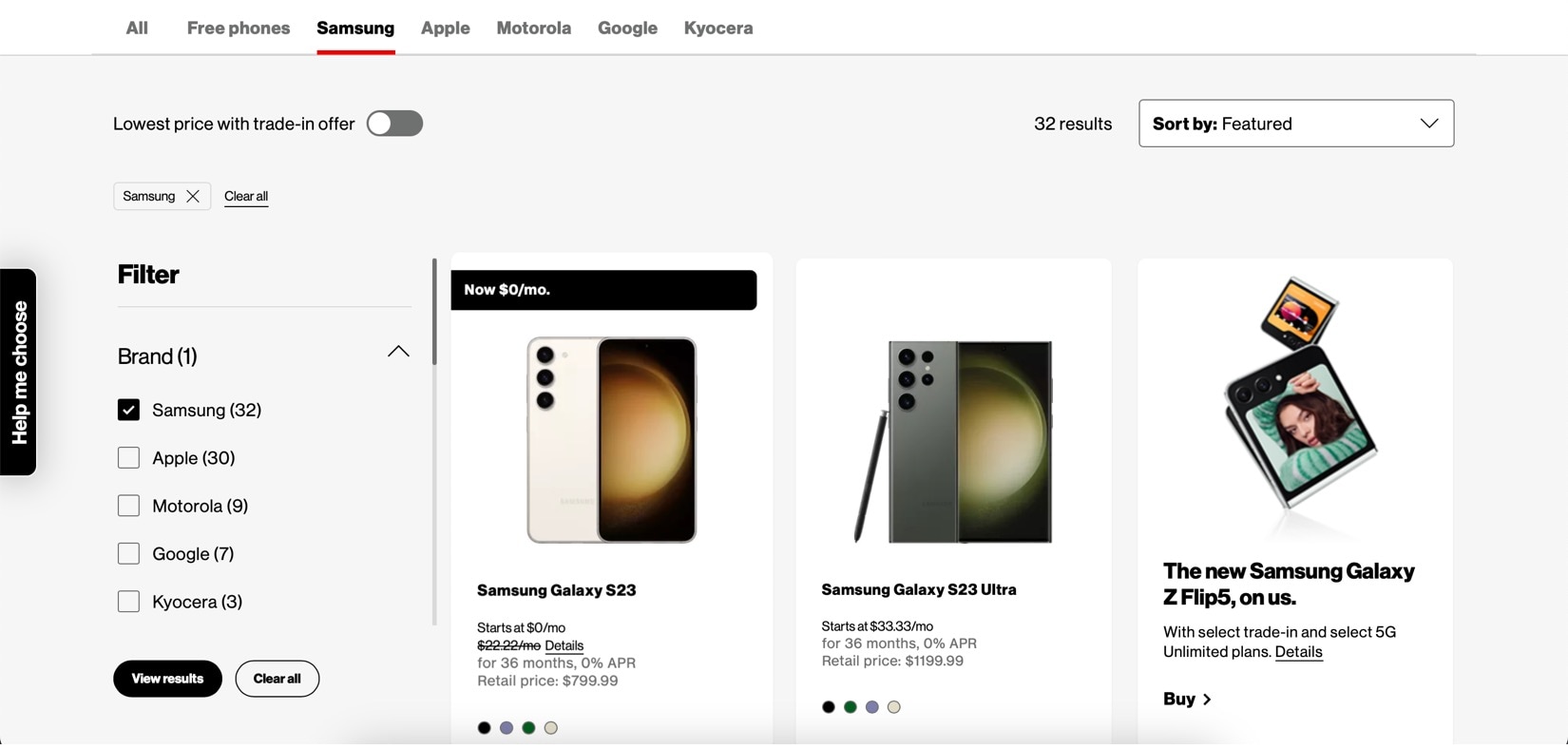The website displays a variety of phones, featuring brands like Samsung, Apple, Motorola, Google, and Kyocera. The user is specifically interested in Samsung phones, highlighted with bold text and a red underline. There are 32 Samsung models available, including the Samsung Galaxy S23, Samsung Galaxy S23 Ultra, and the new Samsung Galaxy Z Flip 5. Each phone is accompanied by a detailed image and specifications.

- **Samsung Galaxy S23**: Starts at $0 per month over 36 months with 0% APR and a retail price of $800.
- **Samsung Galaxy S23 Ultra**: Starts at $33.33 per month for 36 months with 0% APR and a retail price of $1,200.
- **Samsung Galaxy Z Flip 5**: Available with selected 5G Unlimited plans.

Alternative options reveal 30 Apple models, 9 Motorola models, 7 Google models, and 3 Kyocera models.